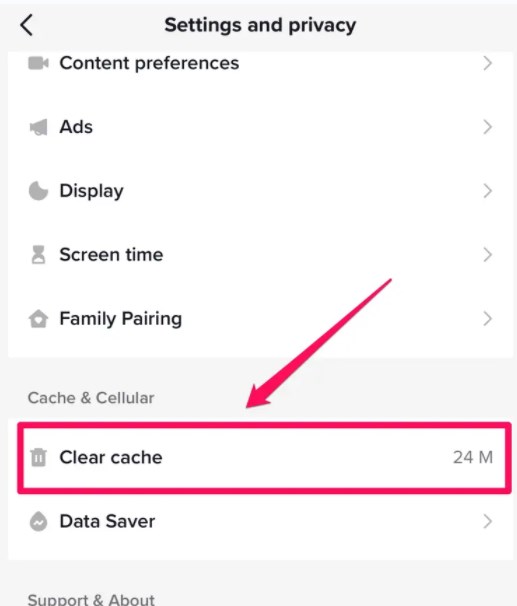The image depicts the 'Settings and Privacy' menu for TikTok, presented in a clean, structured layout. At the very top, there is a gray bar with a list icon on the left, and the title 'Settings and Privacy' centered, all written in black.

Below this header, on a white background, there are several options listed sequentially:
1. **Content Preferences** - Accompanied by a video camera icon.
2. **Ads** - Illustrated with a megaphone icon.
3. **Display** - Represented by a three-quarter moon icon.
4. **Screen Time** - Denoted by an hourglass icon.
5. **Family Pairing** - Marked with a home icon featuring a heart in the middle.

Further down the list:
- **Cache and Cellular** - Noted with an icon of a trash can.
- Below this, the option **Clear Cache**, highlighted by a pink box and arrow. It displays '24M' next to it.
- **Data Saver** - Indicated by a teardrop with a zigzag line through it.
- Lastly, **Support and About**.

All the icons are shaded in gray, while the text for each option is in black. The pink box and arrow pointing to 'Clear Cache' stand out distinctly against the otherwise monochromatic icons, emphasizing the importance of this option.